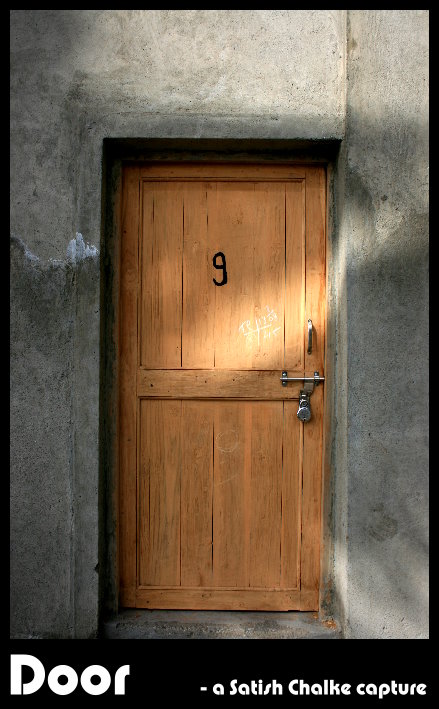The image is a vertically oriented rectangle bordered in black, featuring a photograph of a grey concrete or stucco wall with a centrally positioned wooden door. The door, colored in a distinctive orangey-brown or golden hue, is divided into two panels. In the center of the upper panel, a black marking resembles either the number '9' or a lowercase 'g.' Below this mark, something is scrawled in white, though it remains illegible. The door hardware includes a rustic, drawer-pull style handle situated on the far left, paired with a sliding bar equipped with a silver padlock and deadbolt. The photograph also captures some artistic lighting, with sunlight softly illuminating parts of the door and the surrounding concrete, creating a moody and atmospheric effect. At the bottom of the image, there is a horizontal black bar with white text that reads "door" on the left and "a Satish Chalke capture" on the right.